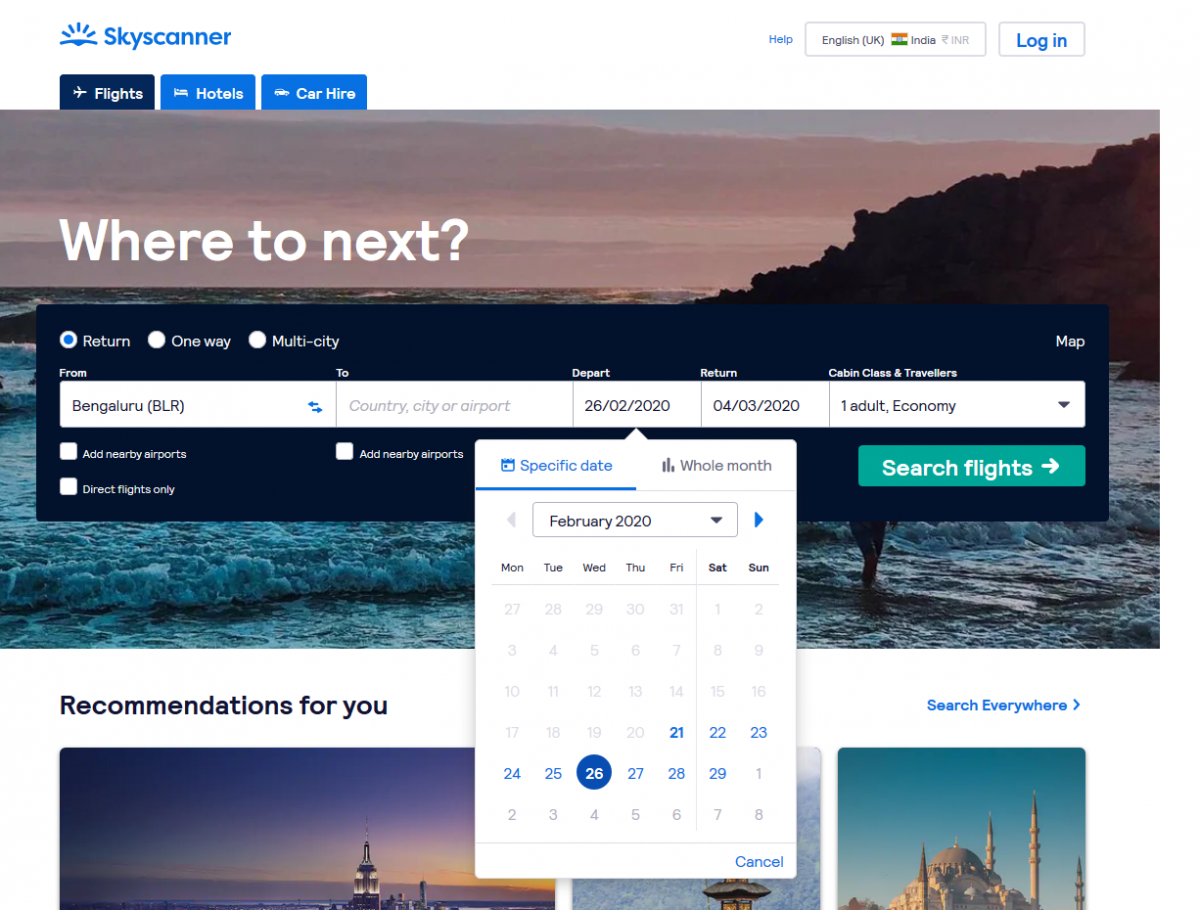In the top left corner of the image, there's a blue "Skyscanner" logo, and the top right features options such as "Help," "English (UK)," the flag of India, and a blue "Login" button. Below the Skyscanner logo, there are three navigation tabs with corresponding icons: a plane for "Flights," a bed for "Hotels," and a car for "Car Hire." The "Flights" tab is highlighted in a darker blue.

The main part of the image displays a scenic view of an ocean area with a hint of mountains in the background, potentially captured near evening. On the right side of the image, a person stands partially obscured by a pop-up window. This window prominently asks, "Where to next?" and features buttons for "Return," "One Way," and "Multi-City" travel options.

Below these buttons are input fields labeled "From Bengaluru (BLR)," "To," "Depart," "Return," "Cabin Class," and "Travelers." The "Depart" section highlights a specific date, February 26, 2020, with an option to select "Whole Month."

Further down, the section titled "Recommendations for You" showcases images of various travel destinations, suggesting options for potential trips.